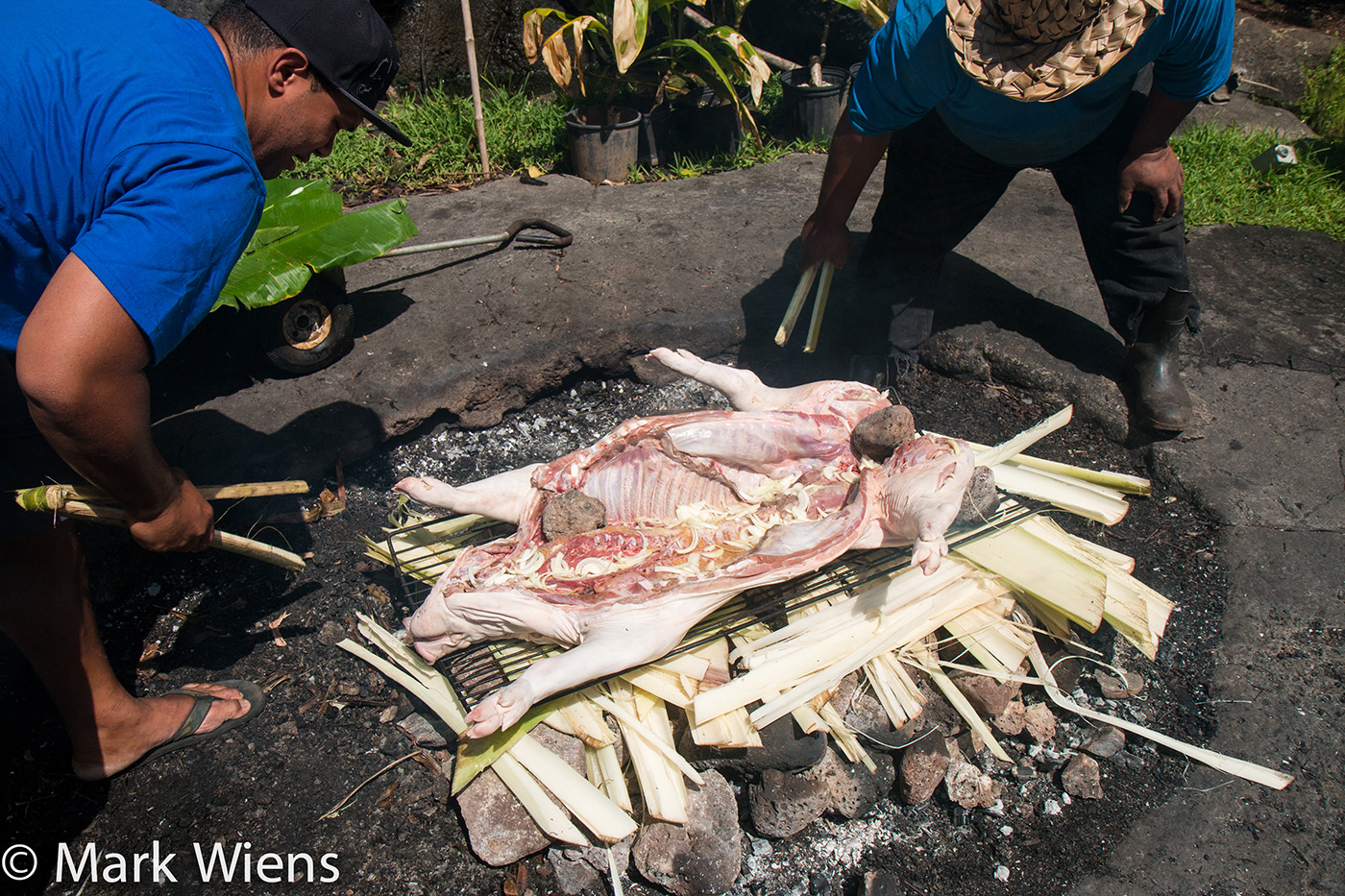This detailed photograph captures an open pit barbecue scene in a tropical outdoor setting, possibly in the Hawaiian Islands, featuring a traditional pig roast. The pig, split open and filleted to reveal its entire rib cage and innards, lies sprawled on a metallic rack. Beneath the rack, green leaves, likely bamboo palms or celery fronds, help support it, while bricks and rocks anchor the structure. Two men, both wearing blue shirts, attend to the roast. The man to the left, dressed in shorts, sandals, and a black baseball hat, seems to be using a palm frond to maneuver the pig. The man to the right, sporting black pants, boots, and a straw-like hat resembling a sombrero, is also engaged in the preparation. They stand on a gray, rocky ground, with tropical plants and grass visible in the background, hinting at the tropical locale. White text in the lower left corner marks the copyright of the image, crediting Mark Wiens.